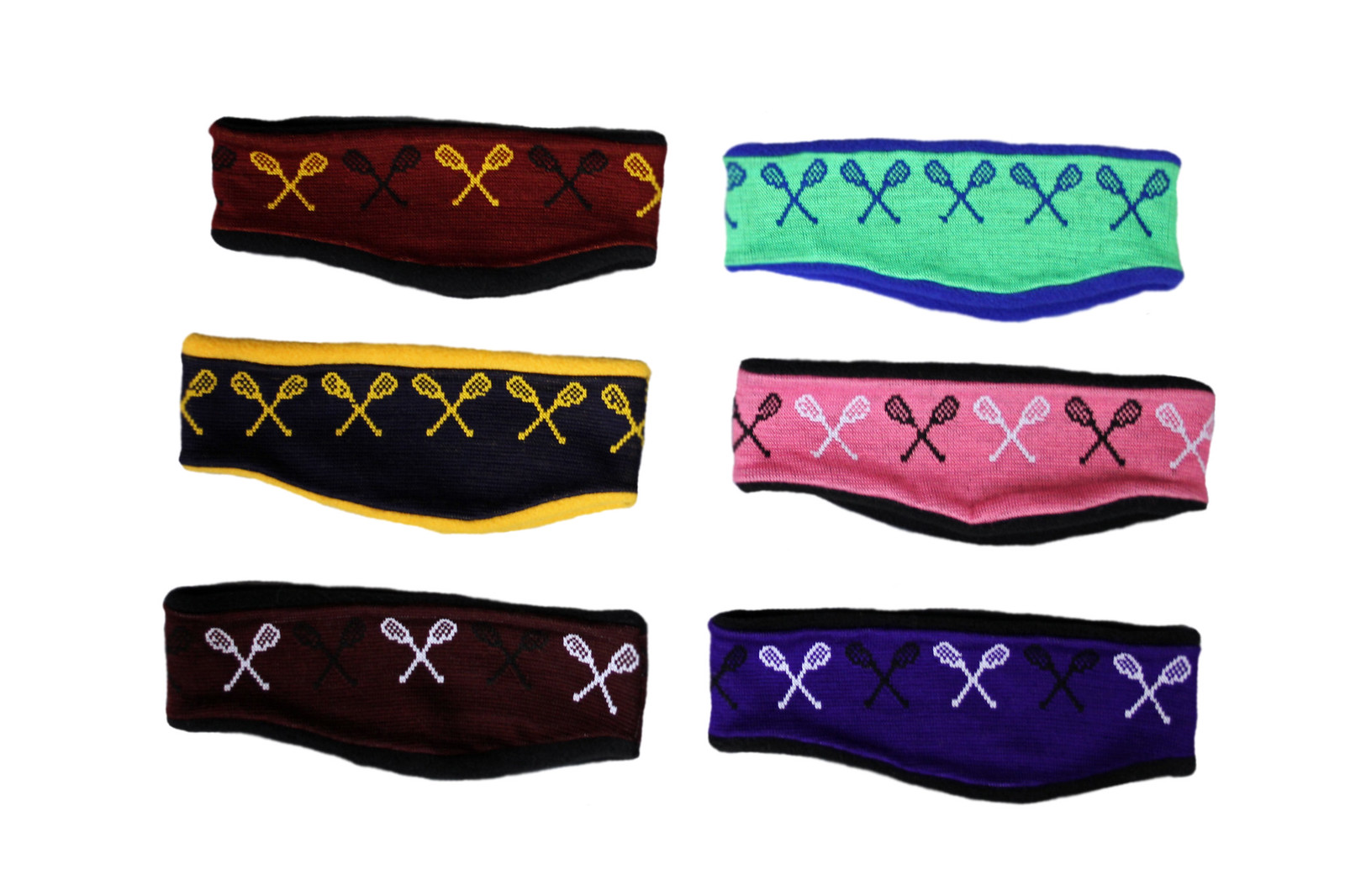The image is a digital photograph with a completely white background, showcasing six headbands arranged in a 2x3 grid. Each headband features a unique pattern that prominently includes lacrosse sticks. The top right headband is primarily a deep shade of red, adorned with alternating yellow and black lacrosse sticks. Next, there is a teal headband with dark blue lacrosse sticks. Then, a darker red headband with yellow lacrosse sticks is visible. A pink headband with varying shades of pink lacrosse sticks follows. The fifth headband is black with light pink and darker black lacrosse sticks that are barely discernible. Finally, the last headband is purple with black and light purple lacrosse sticks. The color schemes and the lacrosse stick designs make each headband distinctive yet part of an apparent set designed for both function and visual appeal.